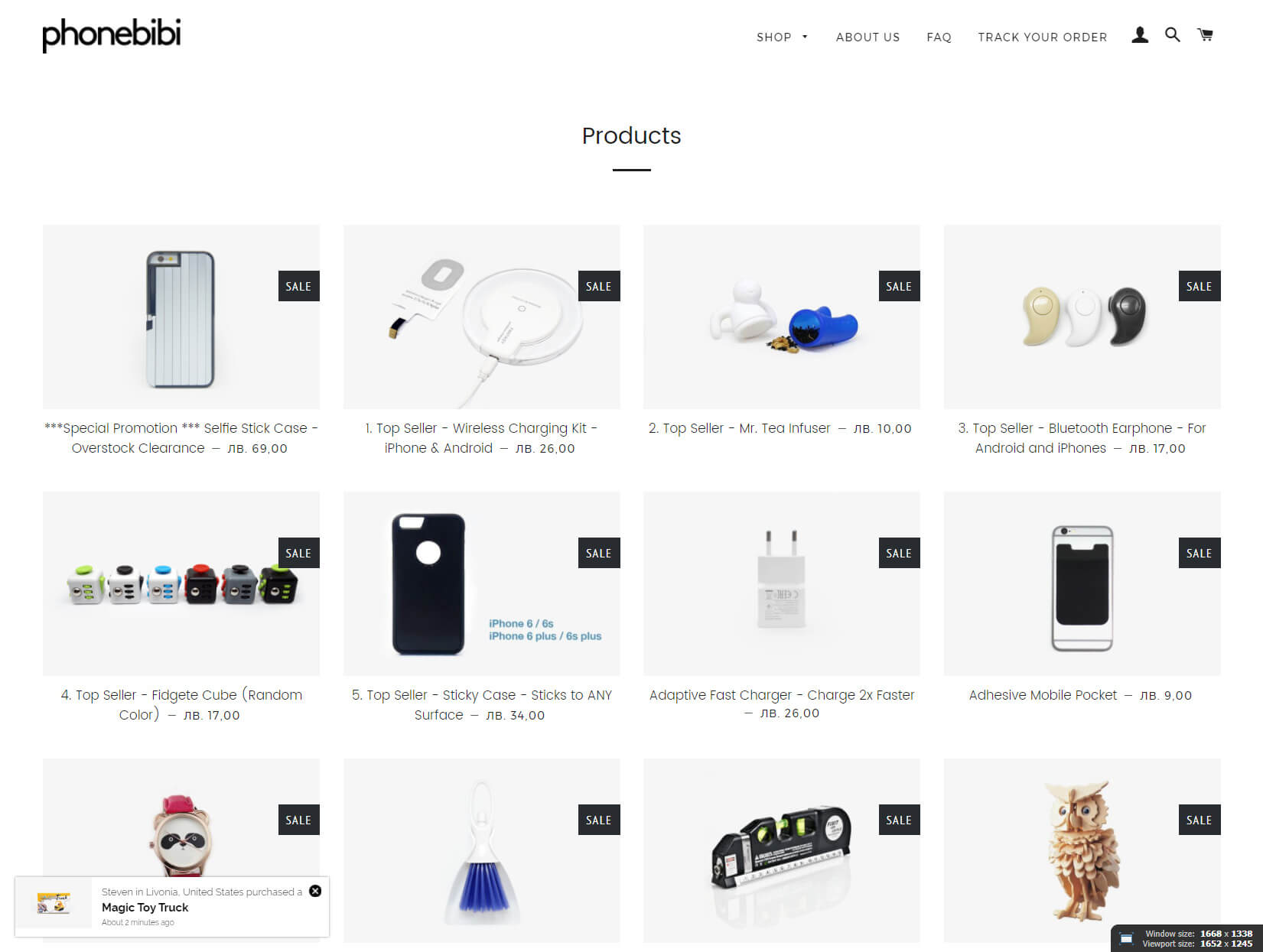The image appears to display a detailed promotional flyer or webpage for various tech and household products. The layout includes several key elements:

- **Top Section:** Features a topless male figure holding a phone on the right side. Beside him, there's a sign that reads "Shop" and various icons including a bodice, a face, a disheveled order, a person, a magnifying glass, and a shopping cart.
- **Headline:** "SALE" is prominently displayed, with a gray background adding contrast. 
- **Starred Promotion:** A highlighted section marked with stars emphasizes a "Special Promotion" for a "Settle Stick Case," part of an "Overstock Clearance" sale priced at $69.
- **Product Listings:**
  1. **Top Seller:** Wireless Charging Kit compatible with iPhone and Android, priced at $26.
  2. **Second Top Seller:** Mr. T Infuser, priced at $10.
  3. **Third Top Seller:** Bluetooth Earphones for Android and iPhone, priced at $17, depicted as teardrop-shaped earphones.
  4. **Fourth Top Seller:** Fridge Cube, available in various colors such as green, black, blue, and red, priced with the description of being a small fridge-like cube.
  5. **Fifth Top Seller:** Sticky Case that adheres to any surface, paired with an adaptive fast charger for rapid charging, and priced to include an adhesive mobile pocket.
  6. **Additional Items:** Features a magic toy truck, a watch, a brush and dustpan combination, a leveler, and a small owl figurine.

This flyer aims to attract attention with its clear organization and prominent promotions.